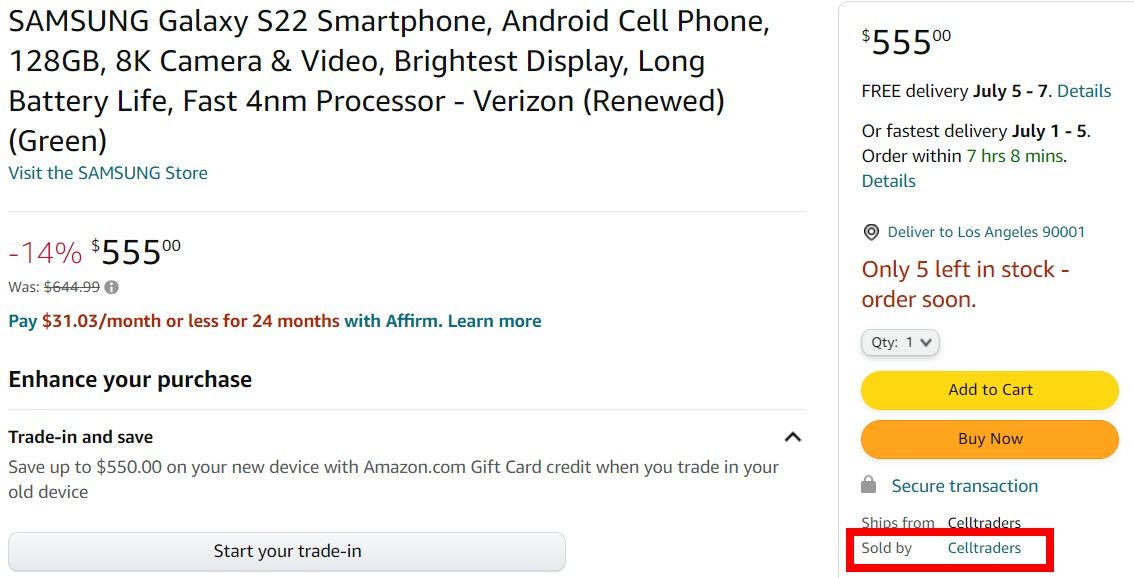**Caption: Detailed Screenshot of Amazon Page for Samsung Galaxy S22**

This image features a detailed screenshot of an Amazon listing for the Samsung Galaxy S22 smartphone. At the center of the attention-grabbing elements on the page is the seller information, prominently displayed as "Sold by Cell Traders" at the bottom right.

Starting at the top of the page, the product is identified as the "Samsung Galaxy S22 Smartphone," further detailed as an Android cell phone with 128GB storage, an 8K camera and video capabilities, the brightest display, long battery life, and a fast 4nm processor. The listing specifies the phone is a "Verizon Renewed" model, highlighted in green.

Beneath this, there's a clickable link saying "Visit the Samsung Store," which directs users to Samsung's store page on Amazon. To the right, typical Amazon purchase options are displayed, including "Add to Cart" and "Buy Now."

The price is stated as $555 with free delivery available from July 5th to July 7th. There's a clickable link for details. The fastest delivery option is from July 1st to July 5th if an order is placed within 7 hours and 8 minutes. The shipping destination is listed as Los Angeles 90001, which is also clickable.

There are only five units left in stock, urging customers to order soon. The quantity can be adjusted from the default of 1 before adding the item to the cart or proceeding to purchase. Below these options, it mentions a secure transaction and reiterates the seller's identity as Cell Traders.

To the left, the price is restated at $555. Payment installment options are available at $31.03 per month or less for 24 months through Affirm, with a clickable "Learn More" link. Below this is an "Enhance Your Purchase" section followed by a "Trade-In and Save" offer. Customers can save up to $555 on their device with an Amazon.com gift card credit when trading in their old device, with a "Start Your Trade-In" link provided.

This screenshot encapsulates all essential elements of the product listing, making it easy to understand the purchase options and offers available.